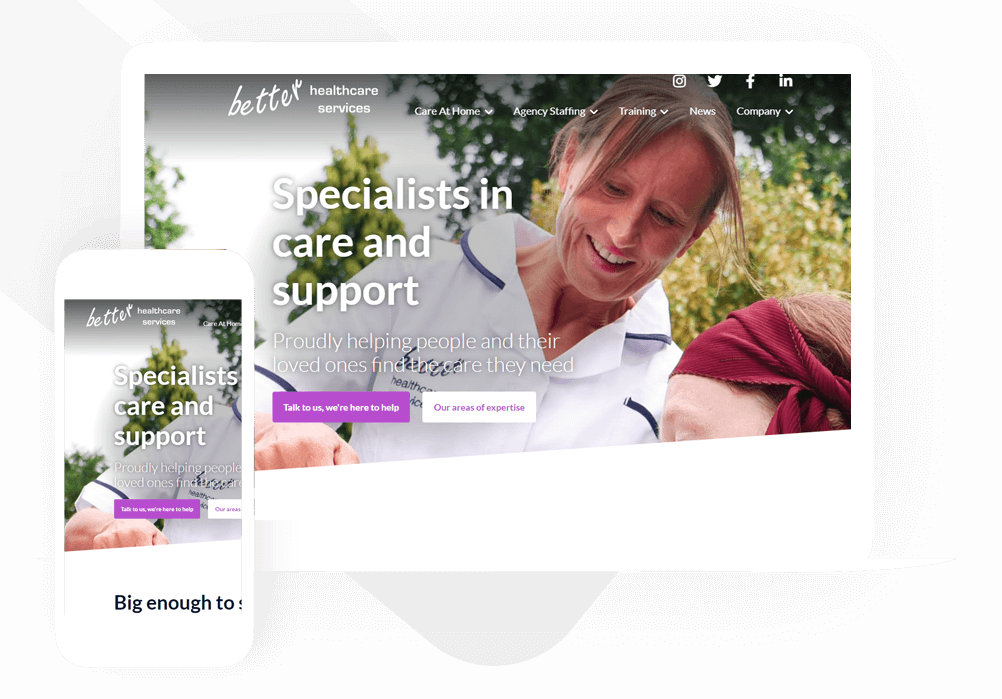The image showcases a website designed for Better Health Services, depicted on a computer monitor with a smartphone positioned at the bottom left corner of the screen. The website's interface includes a dropdown menu featuring links to "Care at Home," "Agency," "Staffing," "Training," "News," and "Company," each accompanied by a downward-facing arrow. Above the menu bar, there are icons for social media platforms including Instagram, Twitter, Facebook, and LinkedIn.

Central to the website is a prominent photograph of a nurse wearing a white and blue uniform, standing next to a person whose head is partially visible, wrapped in a red headscarf. This suggests a focus on personalized care. Behind them, a scenic view of trees is visible, enhancing the serene and supportive theme of the website. A key tagline on the site reads "Specialists in Care and Support," emphasizing the organization's mission to help individuals and their loved ones find the care they need.

Prominently below the image, there are two call-to-action buttons: a purple button labeled "Talk to Us, We're Here to Help" and a white button marked "Our Areas of Expertise" written in purple text. The website's background is predominantly white, and the text is designed to stand out in various colors for emphasis.

The smartphone's display shows a simplified version of the website, with the same background image, tagline, and the purple "Talk to Us" button, although the "Our Areas of Expertise" button is partially cut off due to the screen size.

Overall, the website's design is clean and centered around providing accessible and supportive information for those seeking health care services.